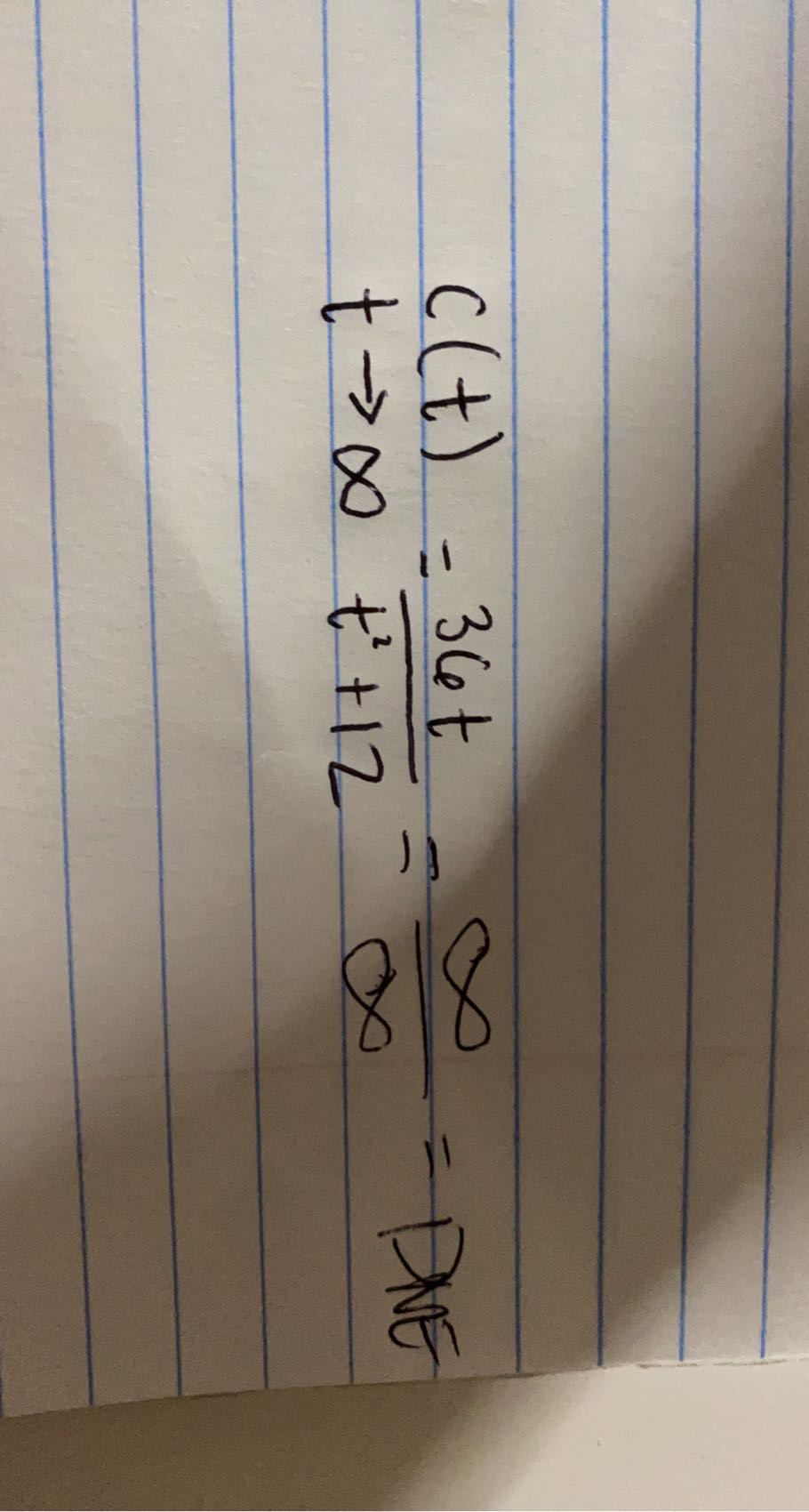A rectangular piece of white notebook paper with thin blue lines, positioned on a flat white surface, is featured in this image. The paper is oriented at an angle, with the top slanting towards the right side of the frame and the bottom leaning to the left. Much of the paper is out of frame, with only a portion visible that showcases handwritten notes in black ink. 

The first line of text reads: 
"C(T) = 36, T = ∞, DNE".

The second line of text features:
"T → ∞, T² + 12 ∞".

A shadow, likely cast by the person taking the photograph, falls over the bottom half of the paper. The shadow extends from the bottom left corner up to the middle right side of the image, partially obscuring some of the handwriting. This likely indicates the presence of the photographer's arm.